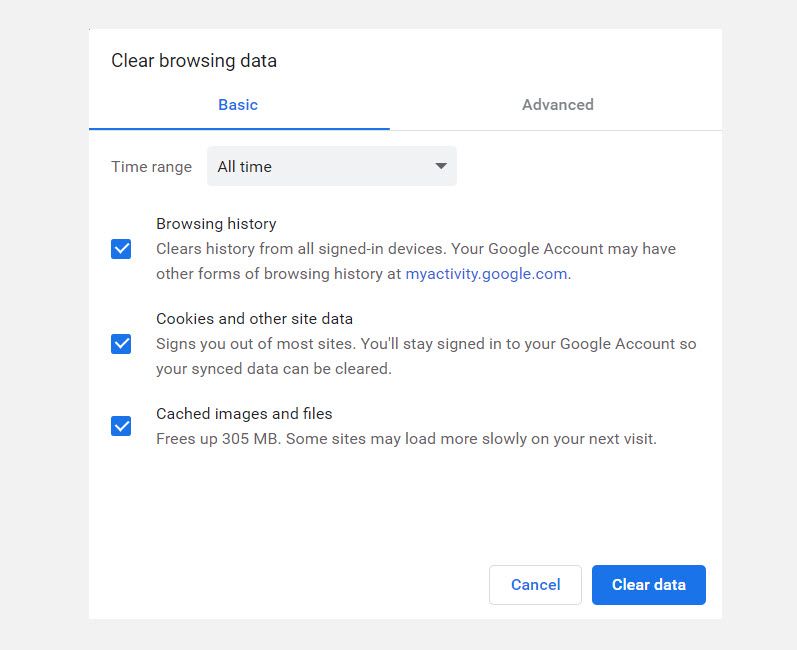The image depicts the "Clear Browsing Data" interface on what appears to be either a Windows device or a Google Chrome browser. The top section of the interface prominently features the heading "Clear Browsing Data." Below this heading, the interface is set to the "Basic" tab by default. In this tab, users are provided with a clickable dropdown menu to select the time range for which they want to delete data. The options available for deletion in the basic tab include browsing history, cookies and site data, and cached images and files. Each of these options is accompanied by a checkbox, allowing users to individually select or deselect the items they wish to clear. To the right of the "Basic" tab is an "Advanced" tab, which likely offers more detailed options for data management, although its specific contents are not visible in the image. This interface provides a straightforward and user-friendly way for individuals to manage their browsing data on their device.